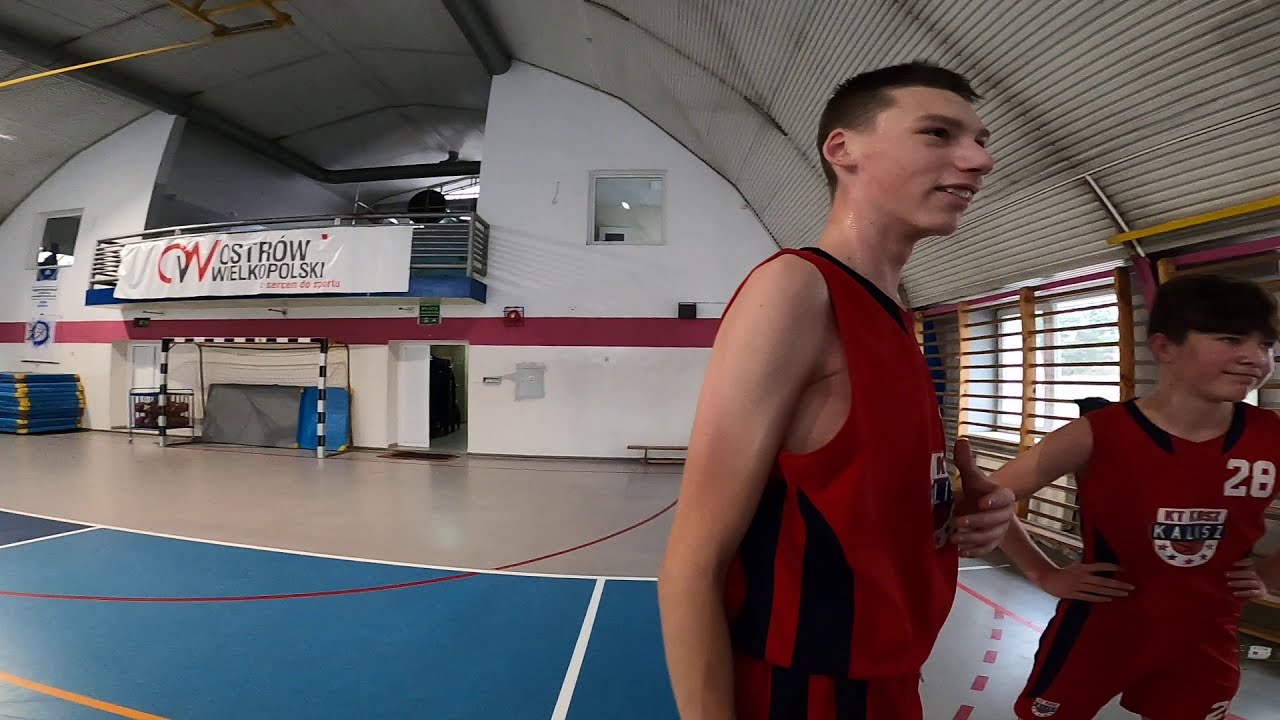The image depicts a scene inside a small gym with an arched white roof and white walls accented by a red stripe. The gym's floor is primarily gray, transitioning to a blue court marked with white and red lines. At one end of the court, there appears to be a soccer net. On the right side of the image are two boys, approximately between the ages of 10 to 14, both dressed in matching red short-sleeve shirts. The boy on the left has a shirt with the number 28 and a white-and-blue logo, while the other boy's number isn't visible. Both boys are smiling and looking off-frame. One appears a little sweaty, suggesting they might have just finished a game or practice. The gym's back wall features a large cutout with a balcony and a white banner that reads "OSTRO-WILKOPOLSKY". The overall atmosphere suggests they are either waiting for their turn or have just completed their athletic activities in an otherwise empty gym.